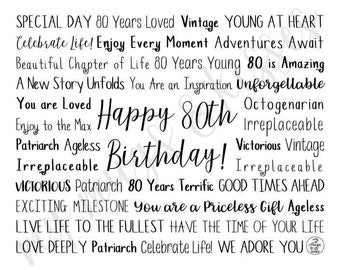The image is a black and white text-based piece in landscape orientation, featuring a celebratory message for an 80th birthday. The background is white with no borders, and the text is arranged in a perfect square alignment. At the center of the image, in large cursive black script, is the message "Happy 80th Birthday." Surrounding this central text, there are about 12 lines of various phrases, each line featuring a mix of different fonts, sizes, and styles including all caps, cursive, and non-cursive.

The text includes heartfelt birthday messages such as "special day," "80 years loved," "vintage," "young at heart," "celebrate life," "enjoy every moment," "adventures await," "beautiful chapter of life," "80 years young," "80 is amazing," "a new story unfolds," "you are an inspiration," "unforgettable," and "you are loved." Additional expressions like "octogenarian," "irreplaceable," "patriarch," "ageless," "80 years terrific," "good times ahead," "exciting milestone," "you are a priceless gift," "live life to the fullest," "have the time of your life," "love deeply," and "we adore you" are also interspersed throughout the design. The eclectic mix of text, fonts, and styles all blend to create a lively and diverse tribute to celebrating 80 wonderful years of life.